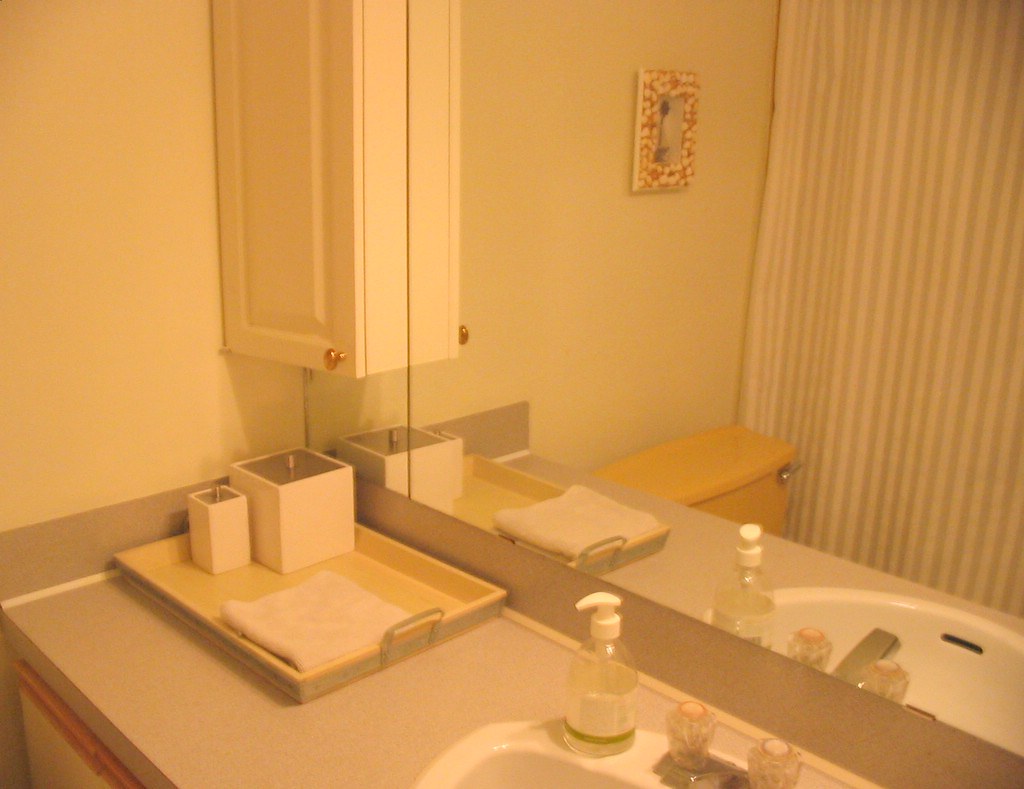This image captures a home bathroom bathed in a warm yellow hue, possibly enhanced by a vintage filter. The overall aesthetic suggests cozy functionality intertwined with a touch of elegance. A large mirror dominates the wall, reflecting the room and revealing additional details. The walls are painted in a very pale medium yellow, creating a soft and inviting atmosphere.

A cabinet, presumably matching the wall color, hangs above the counter with a small gold handle adding a subtle touch of sophistication. The counter space, finished in beige, hosts a neatly organized tray with handles, its interior painted yellow and trimmed with a dash of gray. Two white square boxes, their gray tops hinting at utility for storing items like cotton balls, are positioned on the tray next to a neatly folded towel.

The drawers below the counter are trimmed with wood, harmonizing with the light-colored, perhaps white or pale yellow fronts. The sink area features a double sink with rounded knobs, accompanied by a soap dispenser. A white and yellow striped shower curtain extends across the back of the space, further adding to the room's cohesive color scheme. The toilet, an amber yellow shade, stands out and adds a retro flair. Above it, a picture hangs slightly higher on the wall, contributing a personal touch to this charming bathroom scene.